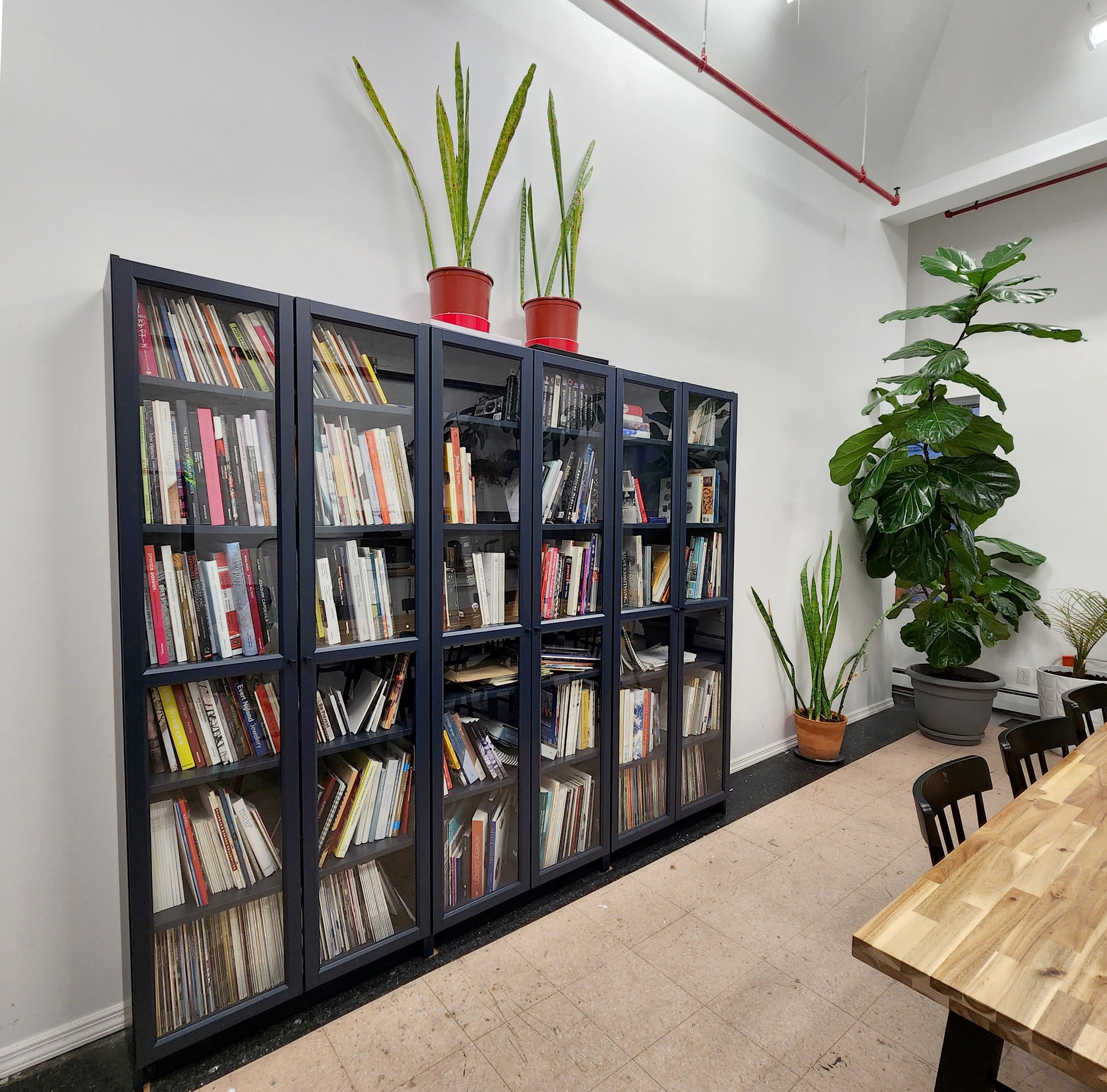The photograph captures a small meeting room or office space with a tall, slanted ceiling and whitewashed walls. In the corner of the room, there is a massive plant in a gray pot, featuring incredibly large green leaves. The black-colored bookshelf, segmented into six glass-paneled cases with six shelves each, is prominently displayed against the left wall, and each shelf is filled with books. Atop the bookshelf, there are two shiny terracotta pots. Against the back wall, a long wooden table with a surface made of different beams of wood is surrounded by black chairs. The flooring is gray tiles, contributing to the room's minimalistic decor. Additionally, thin, orange pipes are held up to the sloped ceiling by strings, and a series of lights hang near the ceiling, offering a functional yet simple atmosphere.